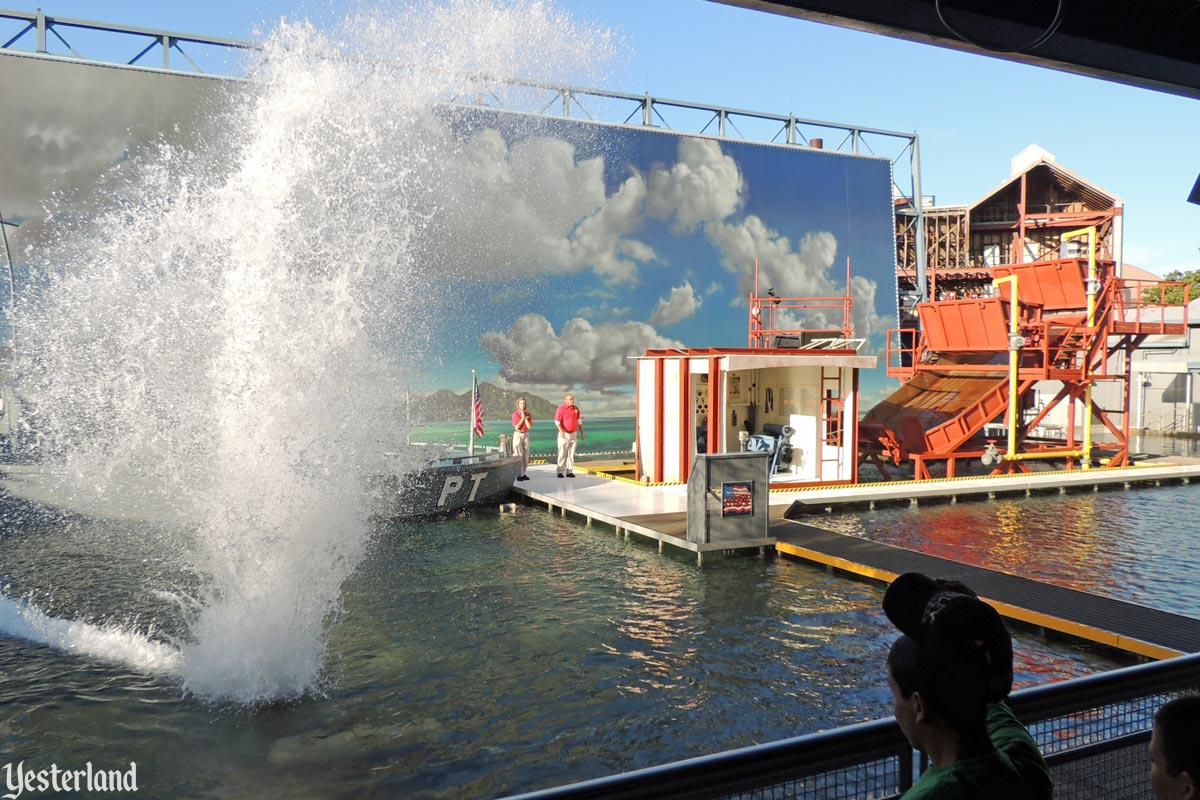The photograph depicts a vibrant scene at what appears to be a themed water park or a historical exhibition area. In the foreground, a group of spectators stands behind a fence, one of whom is leaning over the railing, intently watching the proceedings. Beyond the onlookers, the scene unfolds around a large pond or pool, which is divided into different sections with docks extending over the water.

Central to the image is a significant splash, towering several feet into the air, suggesting that something just fell into or jumped through the water. To the right, there is an orange metallic structure, potentially part of the set, with rust-colored metal girders and panels.

Adjacent to the dock is a gray PT boat, prominently labeled "PT," adorned with an American flag. This placement indicates an evocative historical or theatrical setup, possibly a reenactment of an event such as President Kennedy's time on a PT boat during World War II. Two men, dressed in matching khaki pants and coral polo shirts, stand prominently on a platform beside the boat, perhaps ready to orchestrate the ensuing activity or film a scene.

In the background, a large backdrop frames the scene with a painted depiction of a cloudy sky over an ocean, complete with mountainous islands. Flanking the platform and the PT boat, structures resembling small office buildings or additional staging areas can be seen. It's a clear, sunny day, adding to the lively atmosphere of the park or set. Overall, the image captures a bustling and meticulously arranged setting, teeming with anticipation and historic flavor.